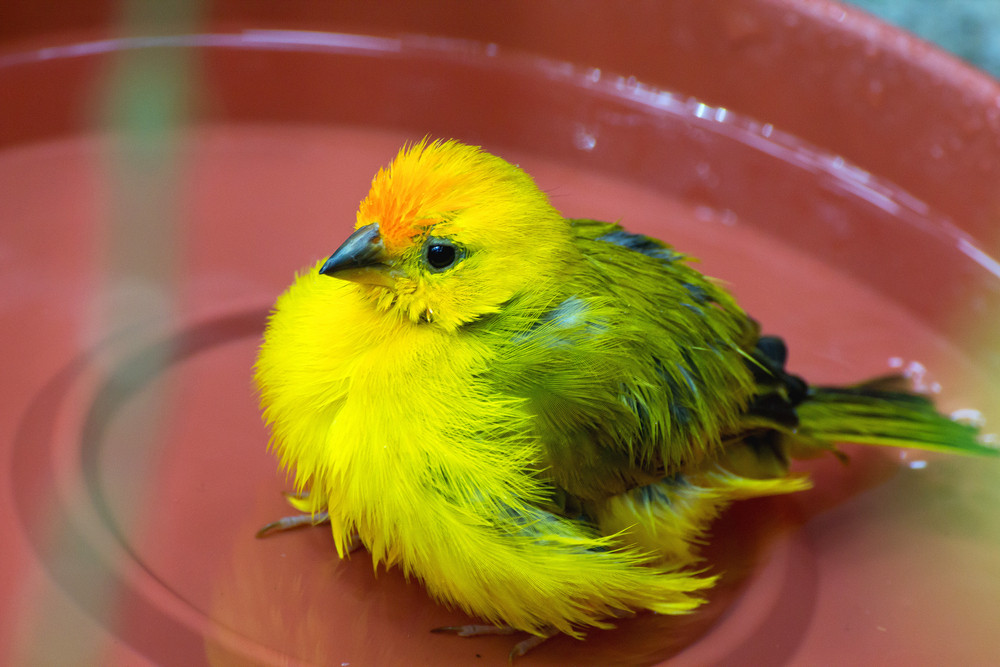A high-quality, professional photograph captures a vibrant, chubby bird in a striking, colorful setting. The bird, primarily yellow with green and dark green feathers, accented by fiery orange on its face and a small black beak, is perched in a shallow, circular, dark red plastic planter dish. The dish, appearing slightly wet as if from recent rain, and the bird's small feet and claws are also visible. Positioned dead center, the bird is seen from its left side with its wings held tight to its body, showcasing its rounded form and vivid plumage. The background is out of focus, emphasizing the bird’s detailed, furry appearance against the multi-colored palette of yellow, green, orange, black, and red, creating a visually engaging and isolated subject with no other animals or people in the scene.